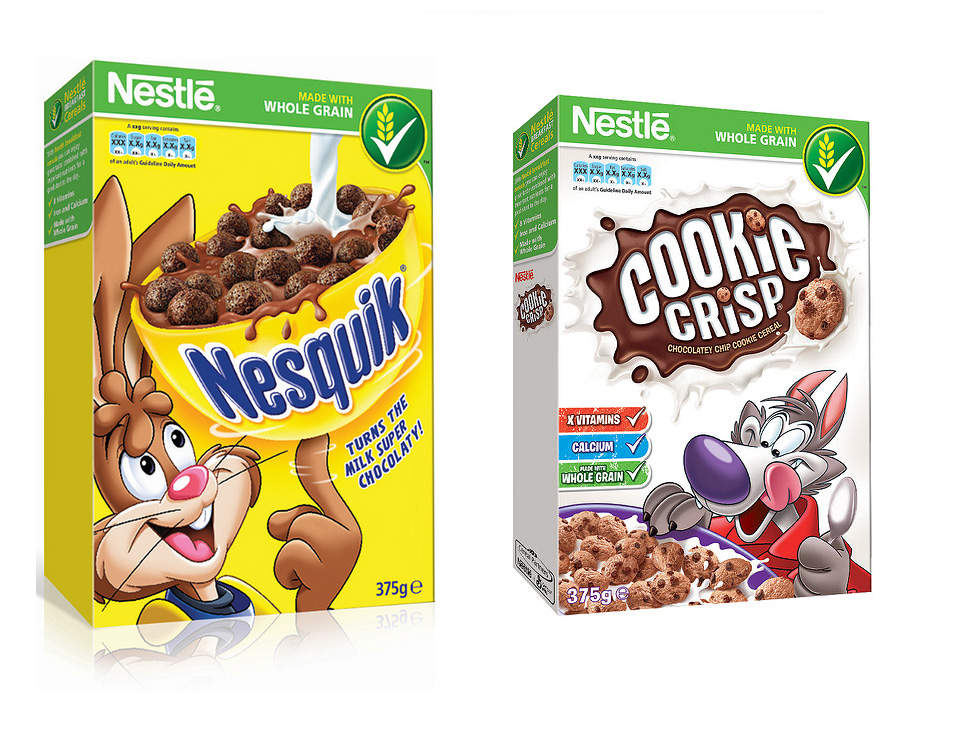This image features a detailed photographic depiction of two boxes of Nestle cereal against a white background. On the left is a predominantly yellow box of Nesquik cereal, accented with a green border at the top. The box showcases a cheerful brown rabbit holding a yellow bowl filled with chocolate cereal puffs. Milk is seen pouring into the bowl, emphasizing the text "Turns the Milk Super Chocolatey!" written in blue. Above the rabbit, the top green border reads "Nestle" in white, followed by "Made With Whole Grain". There’s a graphic of a grain of wheat within a green circle at the far right of the top border.

To the right of the Nesquik box stands the Cookie Crisp cereal box. This box is predominantly white with a green border identical to the Nesquik's, stating "Nestle" and "Made With Whole Grain". The word "Cookie Crisp" is boldly displayed in white with a brown background, complemented by graphics that resemble chocolate chip cookies. The bottom left of the box lists "Vitamins," "Calcium," and "Whole Grain," while the bottom right features a playful wolf, characterized by its purple nose and extended tongue, holding a silver spoon and eagerly eyeing a bowl of Cookie Crisp cereal in milk. Both boxes share similar design elements but feature distinct artwork that highlights their individual cereal themes.